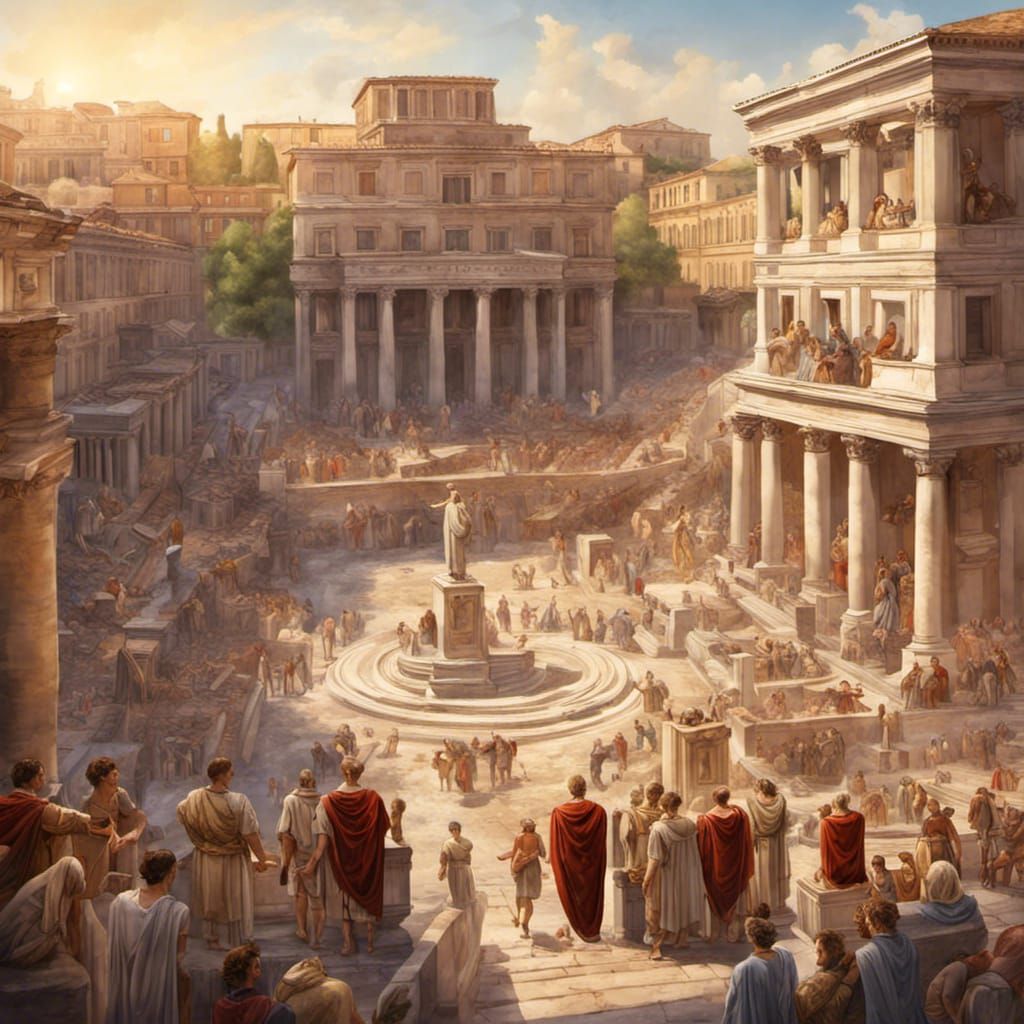This oil painting vividly depicts a bustling scene in ancient Rome. Central to the composition is a grand marketplace or gathering space, dominated by majestic buildings adorned with classical columns. The architectural style is unmistakably Roman, highlighting Rome's grandeur and its citizens' daily life. In the heart of the square stands a prominent fountain, around which throngs of people are gathered. The crowd is diverse, with individuals wearing a mix of red, white, and light blue robes, indicating various social standings and roles within the community. Above it all, the sky stretches out in a serene blue, dotted with clouds, adding to the painting's vibrant atmosphere. This detailed portrayal captures a moment of Roman life, whether it be a regular marketplace scene or an assembly for a particular event, beautifully showcasing the city's historical richness and splendor.